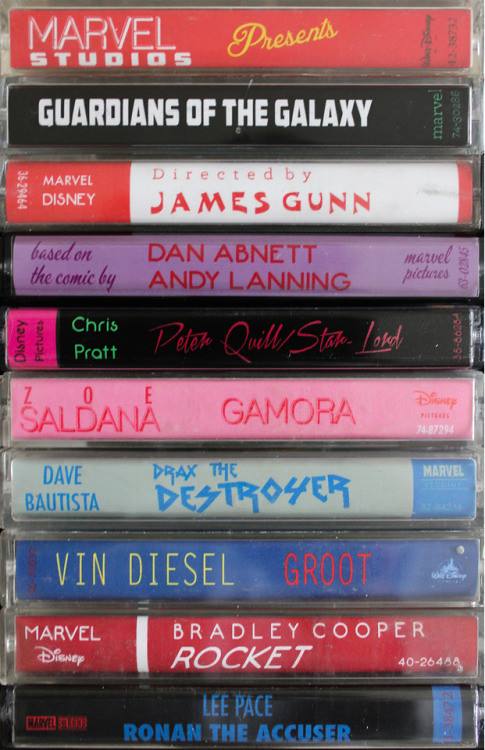The promotional image features a close-up of nine horizontal, colorful cassette tapes, stacked from bottom to top. Each cassette highlights a different aspect of the film "Guardians of the Galaxy" by Marvel Studios, directed by James Gunn. The cassettes showcase notable credits and characters, starting with the bottom one labeled “Lee Pace, Ronan the Accuser” followed by “Bradley Cooper, Rocket,” “Vin Diesel, Groot,” “Dave Bautista, Drax the Destroyer,” “Zoe Saldana, Gamora,” and “Chris Pratt, Peter Quill (Star-Lord).” Additional spines mention “Based on the comic by Dan Abnett and Andy Lanning,” “Directed by James Gunn,” “Guardians of the Galaxy,” and finally, “Marvel Studios Presents.” The cassettes progress in color from red, black, white and red, purple, black and pink, pink, white and blue, solid blue, solid red, to solid black. The overall arrangement creatively mimics classic cassette tapes to promote the film and its ensemble cast.